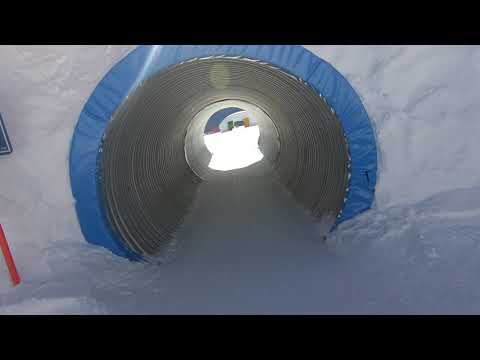In the center of the image, an artificial, reinforced tunnel cuts through a densely snow-covered landscape, flanked by thick snow walls that might extend up to 50 feet high. The tunnel, likely constructed of metal or plastic, features a perfect semi-circular arc and a distinct blue frame around its opening. Its structure is meticulously supported, indicating it was inserted through the snow rather than merely being dug out. The scene is predominantly dominated by shades of white, blue, gray, with hints of orange and red. Outside the tunnel, there is an object on the left side, possibly a shovel or a sign, partially cut off from the picture. The setting appears to be outdoors on a cold, snowy day, adding a stark contrast to the tunnel's structured interior. The tunnel's end is visible, but details beyond are obscured by the snow.